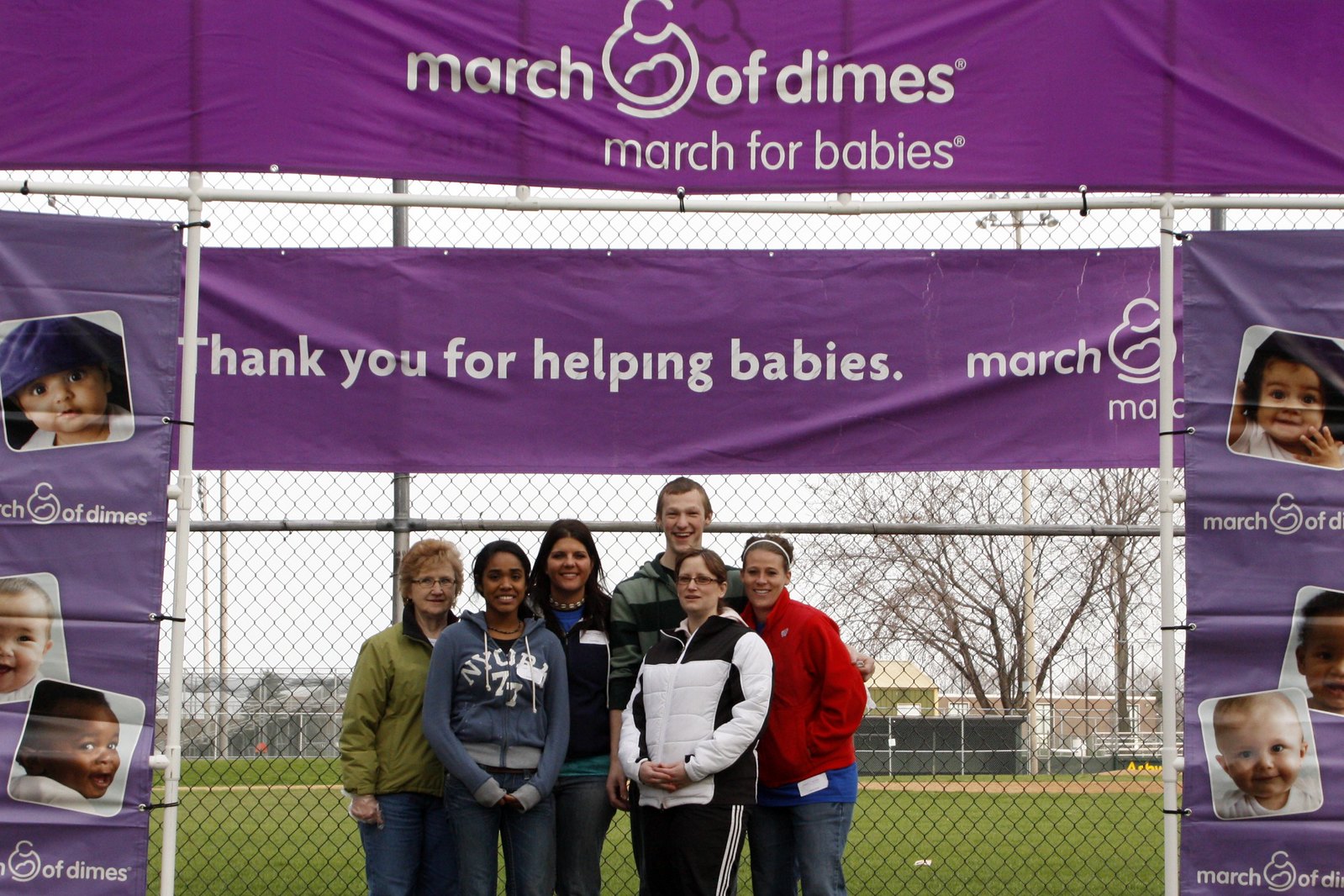In this outdoor image taken at a March of Dimes event, a diverse group of six people are standing in front of a large fence, which encircles what appears to be a baseball field. The fence is adorned with purple banners featuring white text and logos that read "March of Dimes, March for Babies" and "Thank You for Helping Babies." Flanking these messages are multiple images of babies who benefit from the charity's efforts. An overcast sky looms above the park setting, with trees visible in the background, emphasizing a community-centered event on a cool day, as evidenced by everyone's attire.

The group consists of individuals of varying ages and backgrounds, all dressed in jackets appropriate for the weather and wearing event stickers on their clothing. The lineup includes an older woman in her 70s, wearing a green jacket and jeans; a young African American woman in her 20s, dressed in a blue sweatshirt and jeans; a middle-aged Caucasian woman in a dark zip-up shirt over a blue t-shirt and jeans; a Caucasian male in his 20s, attired in a gray striped sweatshirt; a Caucasian woman with glasses, donning a black and white zip-up jacket and matching track pants; and another Caucasian woman in a red zip-up jacket over a blue shirt and denim, topped with a headband. 

All the individuals in the photograph appear happy and engaged, smiling at the camera, clearly delighted to support the charitable cause of helping babies.